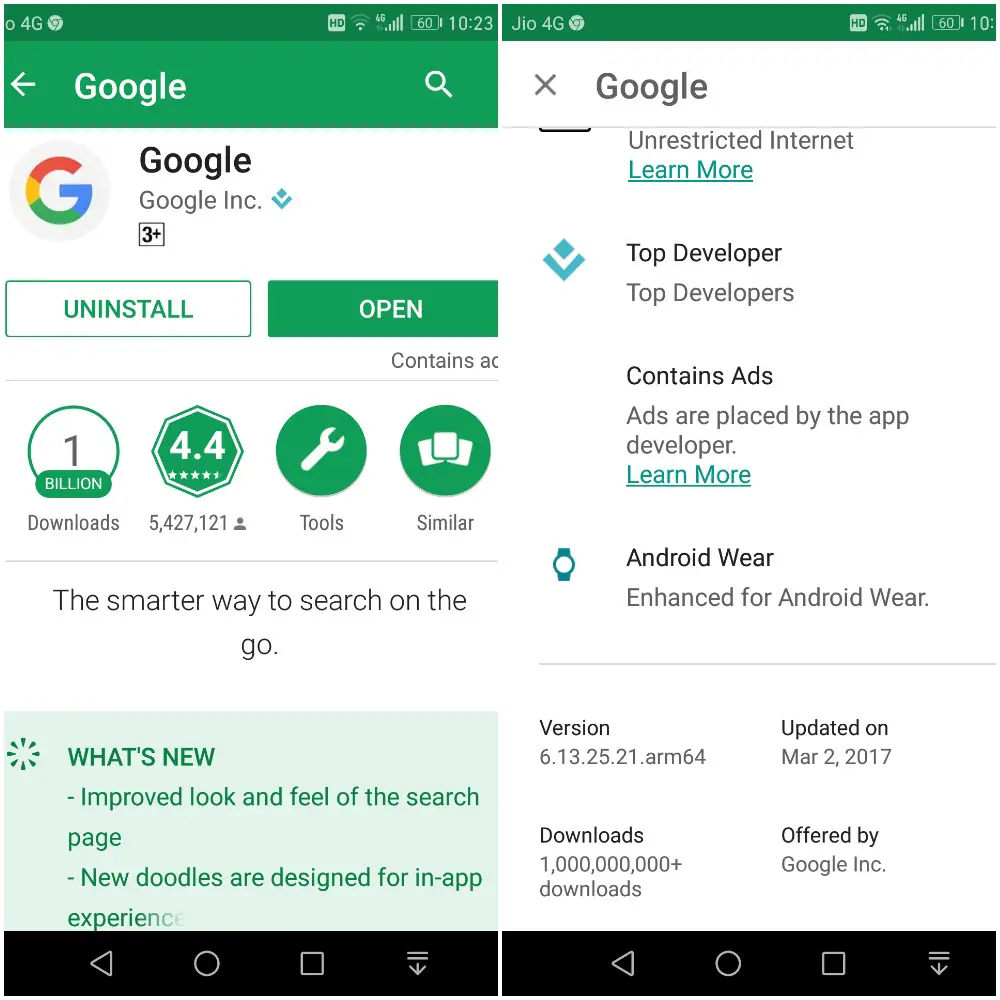The image consists of two screenshots likely taken from a Google operating system device, such as a phone or a tablet. The service provider is indicated as Gio4D, and both screenshots show varying signal strength: three Wi-Fi bars on the right screenshot and two on the left. The device is connected to a 4G network with full signal strength and the battery level is at 60%. The time displayed is 10:23 on the left screenshot, while the right screenshot shows an obscured time starting with "10."

Both screenshots are of the Google Play Store, with the user viewing the page for the Google app by Google Inc. On the left screenshot, you see options to "Uninstall" or "Open" the app, indicating it's already installed. Other details include over 1 billion downloads, a 4.4 out of 5-star rating, and categories such as "Tools" and "Similar apps." The description highlights the app as "The smarter way to search on the go," along with notes on recent updates such as an improved search page appearance and new in-app doodles.

The right screenshot delves into more settings and information about the app. It mentions features like "Unrestricted Internet," "Top Developers," and that the app contains ads placed by the developer. It also notes compatibility with Android Wear and provides details on the current version, which was updated on March 2, 2017. This screen also reaffirms the developer as Google Inc. and the impressive milestone of over a billion downloads.